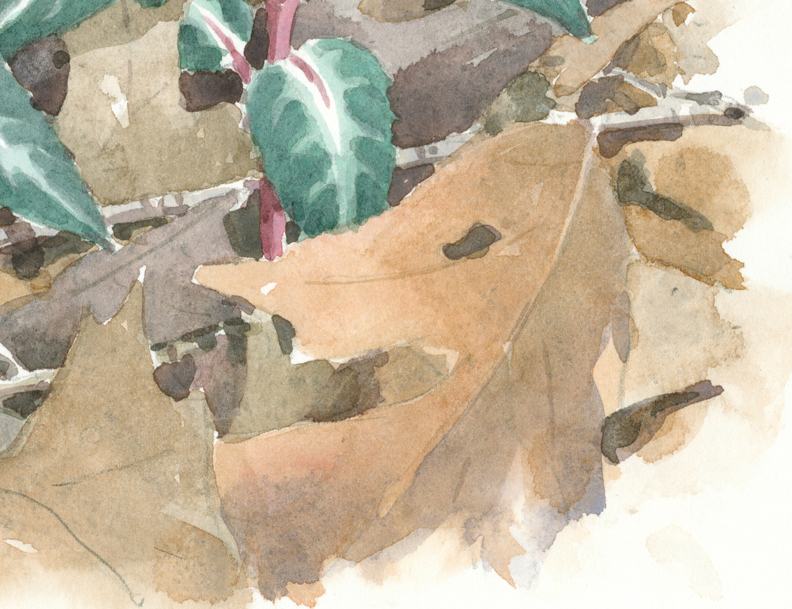This is an artist's detailed rendition of a pile of leaves, predominantly in shades of brown, with a few green and purple elements adding contrast. The painting, which may be watercolor, digitized, or oil-based, features a large light brown leaf prominently in the foreground, accompanied by another brown leaf and a green one. Interspersed among the leaves are some twigs, suggesting they may still be attached to branches. A striking red stem or vine grows through the center of the composition, supporting vibrant green leaves with red veins. The background is mostly white, visible primarily on the right side and the lower right corner, where the leaves are less dense. There may also be a small drawing of what could be a beetle among the leaves. The style captures the essence of autumn with its depiction of dried, slightly torn leaves and the contrasting lively green foliage of the stem.